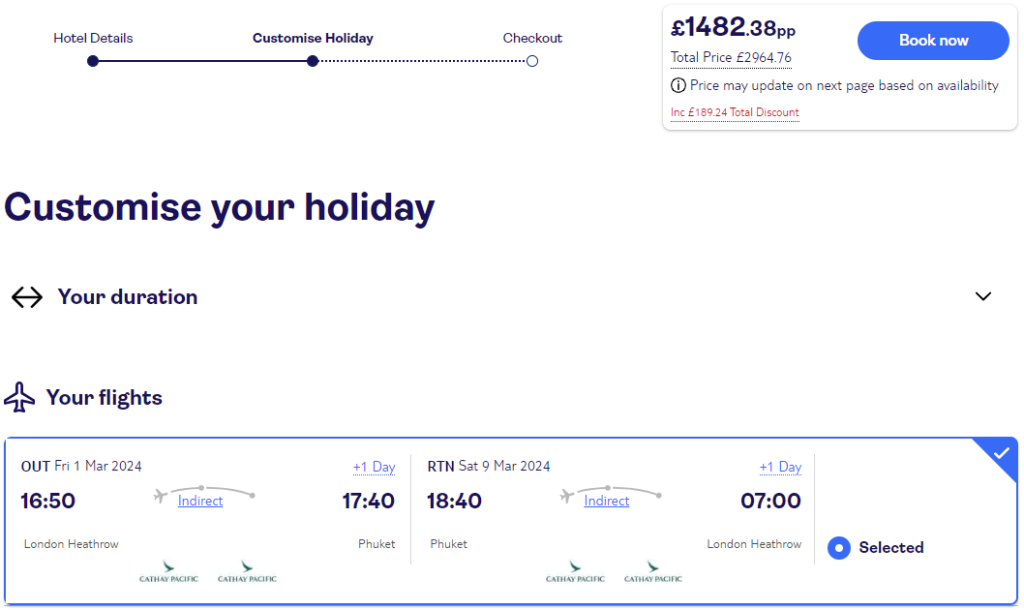The image depicts a section of an order screen for booking a holiday, with a three-step process displayed at the top left corner. The steps are as follows: 
1. Hotel Details (checked off)
2. Customized Holiday (highlighted as the current step)
3. Check Out (not yet completed)

The background of the screen is white. On the right side, there is a box showing the value "1,482.38 pounds", and the total price is prominently displayed as "2,964.76 dollars". Below the price details, there is a "Book Now" button, followed by sections for customizing the holiday's duration and flight details.